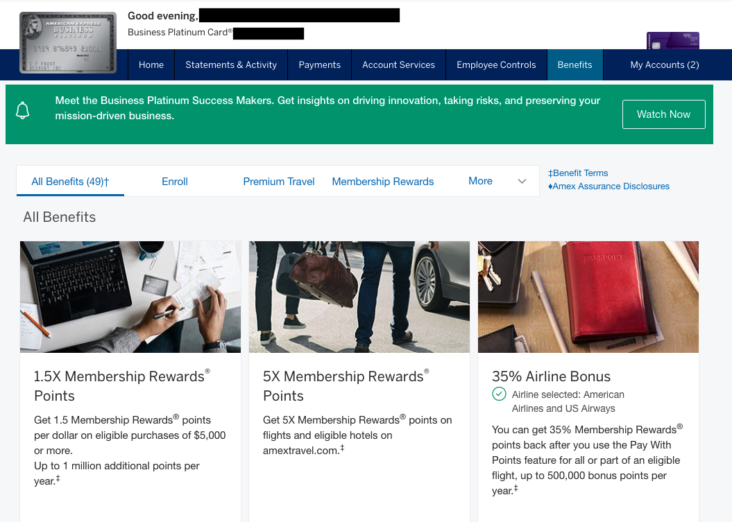The image depicts a banking website interface, evidently designed for business account management. At the top right corner, there's a section labeled "My Accounts," with the number "2" indicated in parentheses. Moving left along the top menu, the options displayed include "Benefits," "Employee Controls," "Account Services," "Payments," "Statement," "Activity," and "Home." 

Adjacent to the "Home" button, there's a high-resolution image of a silver credit card embellished with a Roman-style icon on the top left corner. To its right, the greeting "Good Evening" followed by the title "Business Platinum Card" is clearly visible. Further to the right, there's a black obscured area, possibly redacting sensitive information.

Centered at the top of the page, a promotional banner reads: "Meet the Business Plan of Success Makers: Get insights on driving innovation, taking risks, and preserving your mission-driven business." Beneath this banner, several categories are listed, including "All Benefits," "Enroll," "Premium Travel," "Membership Rewards," and "More" in light blue text. "All Benefits" stands out, highlighted by a dark blue underline, suggesting it is currently selected.

The bottom half of the image features three separate pictures. Above the first image, a caption reads "All Benefits." The first picture promotes "1.5X Membership Rewards," the second touts "5X Membership Rewards," and the third highlights a "35% Airline Bonus."

This detailed and organized layout indicates the website’s aim to provide comprehensive banking and rewards management services for business account holders.